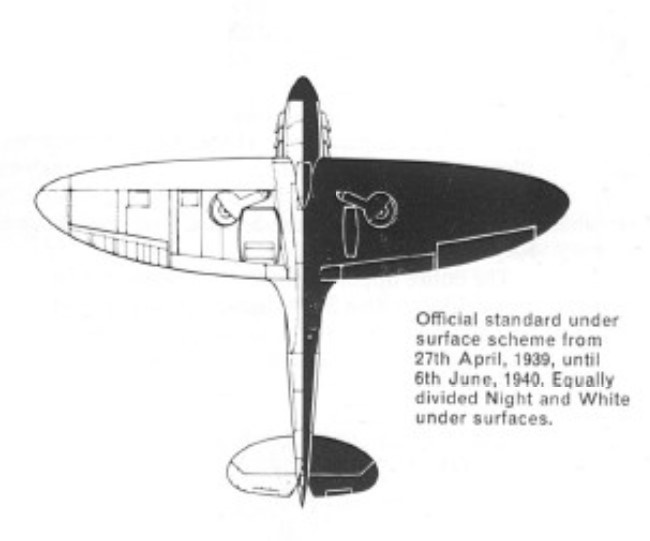The image is a somewhat blurry, hand-drawn sketch of an early model airplane viewed from above. The design is symmetrical, with the left half of the airplane shown in white with black line details, and the right half in black with white line details. The airplane's design appears rudimentary, reminiscent of a surfboard in shape, with simple left-and-right extending wings and a horizontal tail fin at the back. In the lower right corner, there is a text that reads: "Official Standard Under Surface Scheme from 27th April 1939 until 6th June 1940, equally divided night and white undersurfaces." The overall sketch is monochromatic and has a white background.